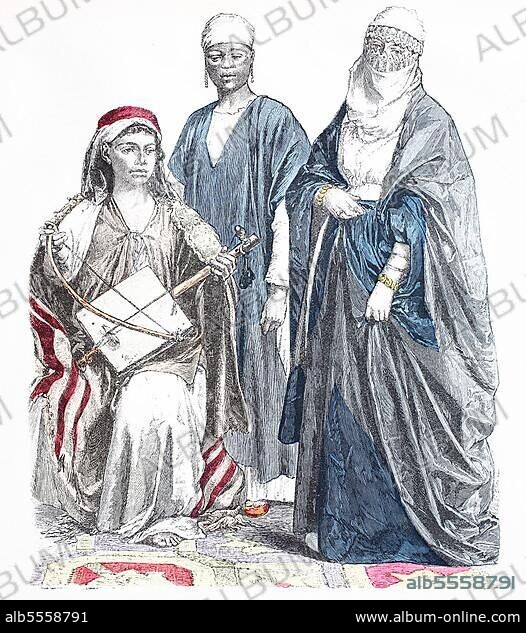The vertically aligned rectangular image, resembling a stock photo, features a finely sketched drawing of three women, set against a white background with the word "ALBUM" repeatedly printed diagonally in gray, all caps. The woman on the left is seated, adorned in gray and white attire with a red hat, and she's holding an object that appears to be an ancient violin or some sort of musical device. The central figure, standing, dons a blue gown with a gray wrap and appears to have an African feature. She seems to have a banner draped behind her in red and light gray, extending over her head. The woman on the far right is also standing, enveloped in a blue gown and gray wrap, her face completely covered except for her eyes. In the lower right corner, the code "ALB555879" is displayed in green, and at the bottom, a black border bears the text "ALB5558791" in white on the left side and "www.album-online.com" on the right. Also, there is a small brown wedge at the bottom center, potentially depicting the central woman's foot.